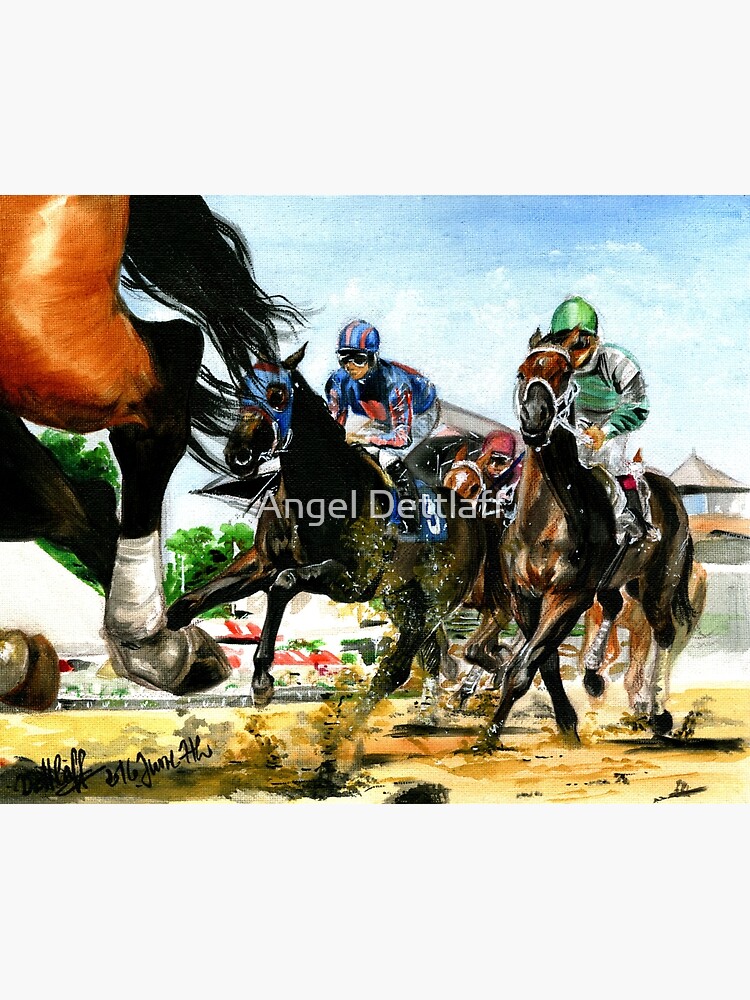This painting by Angel Detlef vividly captures the dynamic and thrilling atmosphere of a horse race from a unique angle. The scene showcases four galloping horses on a dirt track, with disturbed soil visible beneath their powerful strides. In the foreground, the hind legs of a chestnut brown horse with a black tail and hoof, and a hint of white on its foot, are prominently displayed. Behind this horse, three riders are in focus, each donning distinctively colored uniforms: one in blue with a matching blue mask and saddle, standing tall on his horse; another in green; and a third partially obscured rider in red. The backdrop reveals distant box seats for spectators beneath a bright blue sky, flanked by trees to the left, completing the lively depiction of the race. Detlef's signature is subtly signed in the bottom left corner, marking this intricate and engaging piece.